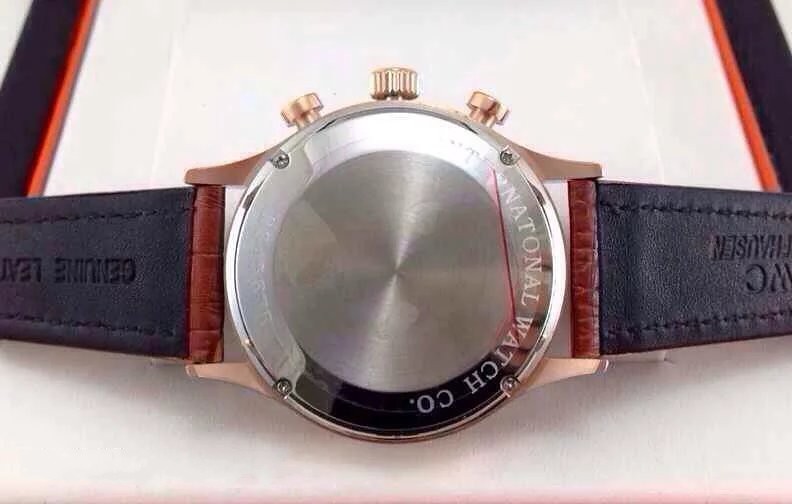A detailed image of the back of a wristwatch, prominently displayed on a white, plush surface. The watch is framed by a striking black and red border on both the left and right sides. The bottom strap of the watch is black leather, meticulously detailed with stitching. The left strap explicitly indicates it's made of "genuine leather." Meanwhile, the right strap features the partial letters "WC," with the remaining characters indiscernible. Notably, the area where the strap connects to the watch case is composed of brown leather. The watch case itself combines gold accents along the outer edge with a silver back, which bears the engraving "International Watch Company."